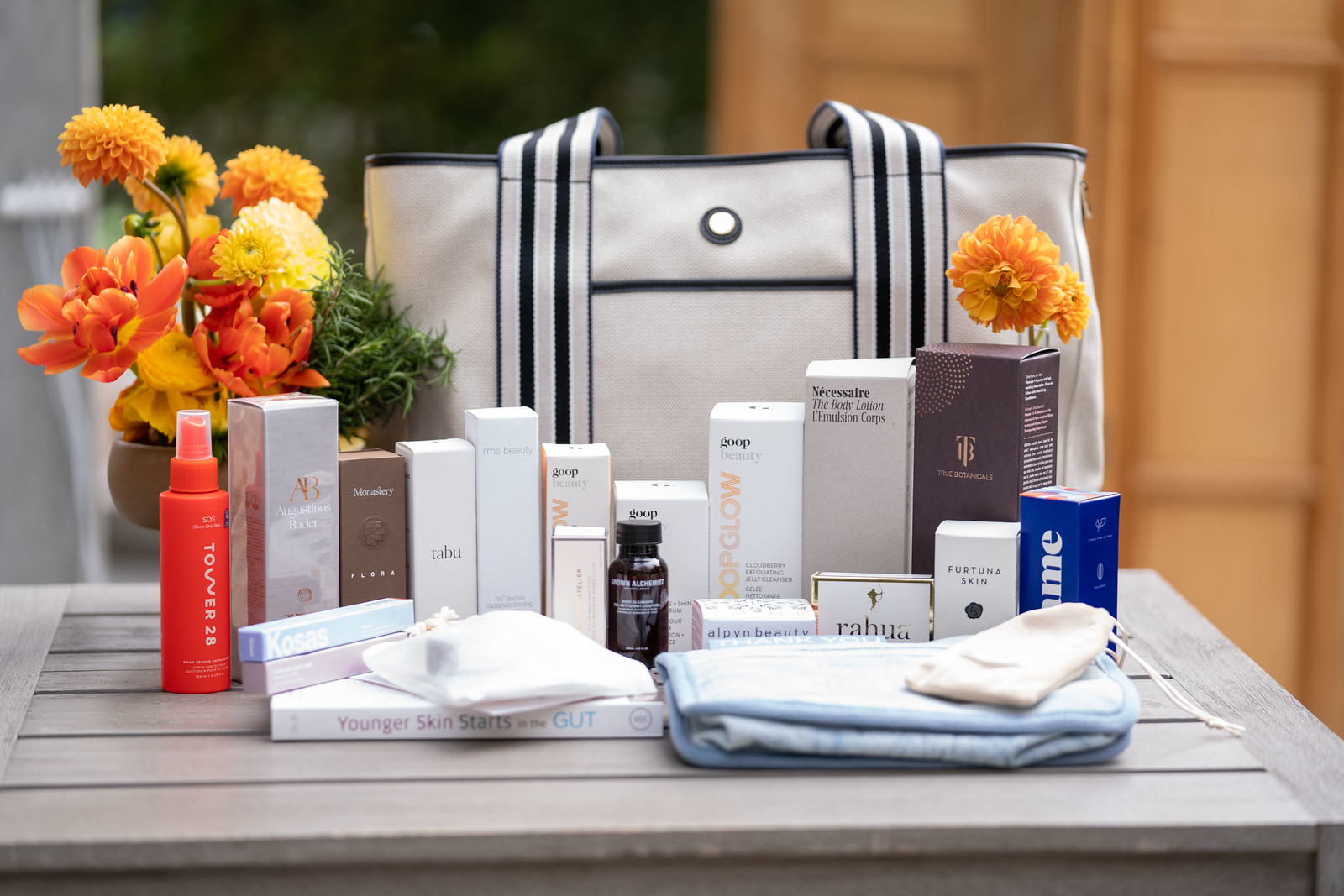The image depicts a gray patio table with wooden slats, neatly arranged with an extensive collection of beauty items, including makeup, spritzers, moisturizers, and various skincare products. Prominently placed on the table is a white book titled "Younger Skin Starts in the Gut." To the right of the book lies a blue towel, topped with a small white drawstring pouch. Behind these foreground items, there is an organized array of boxes, spritzers, and vials. The collection includes an orange box among other packaging in shades of gray, brown, cream, off-white, and blue. Adding a touch of nature, a flower vase with bright yellow flowers is positioned in the back left, complemented by a single yellow-orange flower on the right side of the table. In the background, a gray bag with black accents suggests it originally held all these beauty products.